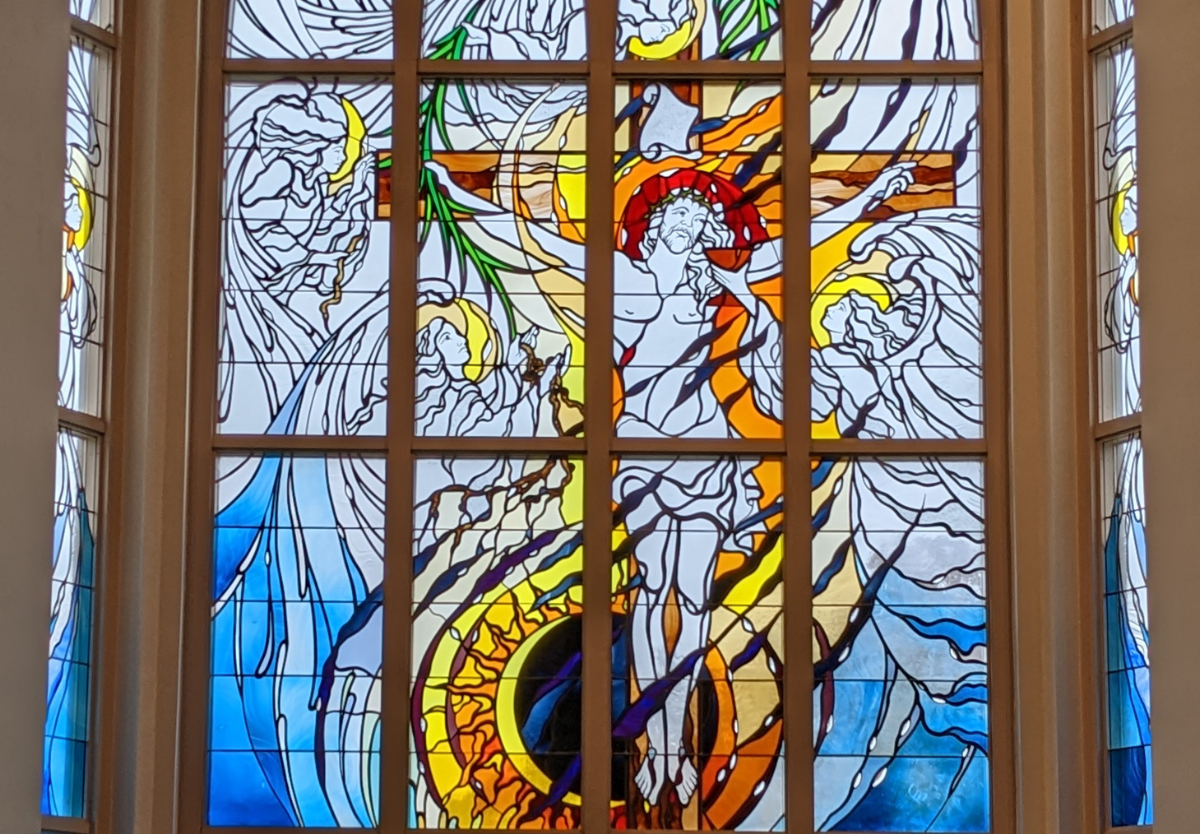The image is an intricate stained glass window of Christ being crucified, comprised of multiple wooden-brown panels that frame the composition. In the center, Jesus' solemn face is surrounded by rich red stained glass panels, while the rest of His body is depicted in light gray hues. Dark blue streaks pierce through His body and legs, adding dramatic contrast. Surrounding Him, there are angels with expansive, flowing wings, which meld into blue patterns that resemble the sea. One angel is presenting an orange-colored cup to Christ's face, while another, on the left, holds up her hands with a brown string dangling from them. There is an angel above, adding to the heavenly scene. Above Christ's head, a scroll is depicted, and beneath His feet lies an enigmatic image of an eye, possibly signifying an eclipsed sun. Green palm fronds also feature in the design. Wooden frames encase this vivid portrayal, and additional fragments of stained glass adorn the walls adjacent, hinting at the surrounding sacred space. This evocative artwork, likely housed within a church, stirs emotions of sorrow and gratitude.